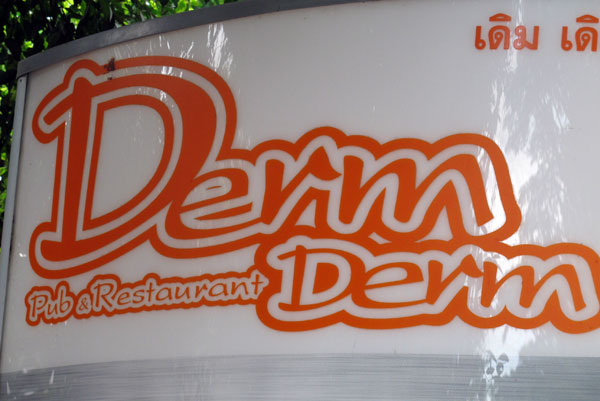The image showcases a tight close-up of an outdoor street sign for a restaurant named Derm Derm. The sign features glossy, reflective glass that reveals subtle reflections of surrounding trees. In the top left corner, dense, dark green vegetation is partially illuminated by light peeking through. The sign prominently displays the name "Derm" in a large, curvy, stylistic orange font with a white outline and an additional orange outline. Below, in much smaller text, it reads "pub and restaurant," and to the right of this is another instance of "Derm." The sign appears to be designed to light up, possibly indicating built-in lighting for nighttime visibility. Additionally, the top right corner of the sign contains text in a foreign language, hinting at a Southeast Asian locale, further contributing to its distinctive aesthetic.